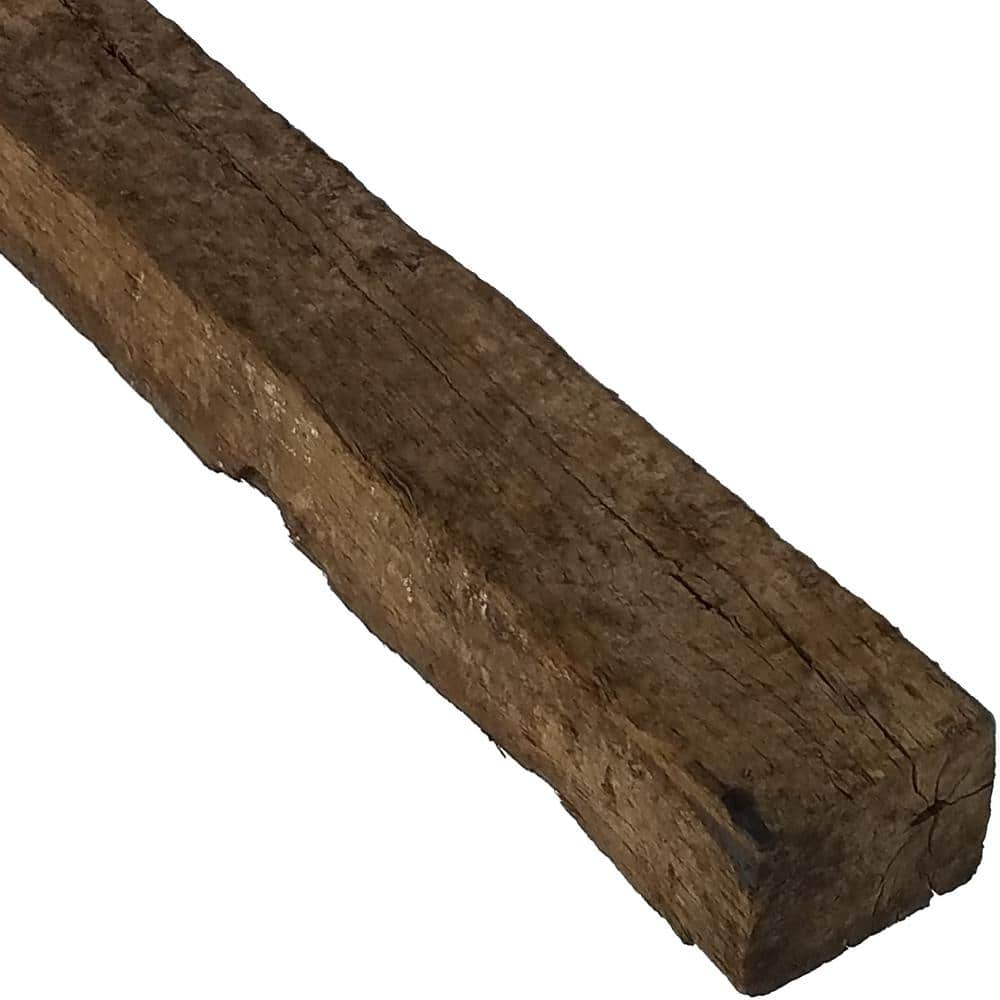This highly detailed close-up photo features an aged, weathered wooden beam prominently set against a completely white background, resembling a product display. The wood, appearing to be a 2x4 or 4x4 shape and a mix of various shades of brown and black, is in a state of visible distress and damage. Deep, extensive cracks run along the length of the beam, adding significant texture. Multiple sections of the wood show missing chunks and flaking, with noticeable pitting and indentations—particularly a circular crack at the bottom that's spider-webbing outward. The top of the beam is especially stressed and cracked, while the left side reveals additional missing pieces, possibly from rot or damage. Notably, sun-like rays of cracking can be seen emanating from small holes, particularly in the right-hand corner, emphasizing the beam's extensive aging and degradation. Despite its decrepit state, the beam's detailed portrayal against the stark white background evokes a sense of its history and long-term wear and tear.